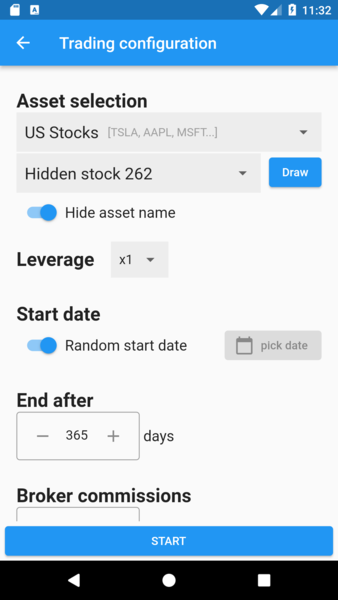This image is a detailed screenshot of a trading app interface. The topmost section features a blue header displaying the text "Trading Configuration," with indicators showing the screenshot was taken at 11:32 AM and the cell phone battery is fully charged at 100%. 

Beneath the header, the app's main body has a clean design with a white background and black text. The first section, labeled "Asset Selection," includes a drop-down menu set to "US Stocks" (TSLA, AAPL, MSFT).

Below that, there is another drop-down menu displaying "Hidden Stock 262," accompanied by a blue "Draw" button to its right. Beneath this menu is a toggle button that is switched to the "on" position, highlighted in blue, and labeled "Hide Asset Name."

Further down, the app provides a section for setting leverage, with a drop-down menu currently set to "1x." 
The next parameter is the "Start Date" setting, which has a toggle button also set to the "on" position for "Random Start Date," alongside a clickable box to manually select a start date if desired.

The "End Time" setting is configured to 365 days. The section labeled "Broker Commissions" sits below, though its details are not fully visible in the screenshot.

At the bottom of the interface, a prominent, long blue "Start" button is present, ready for user interaction.